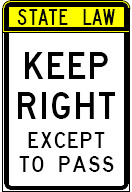This image features a road sign designed to communicate traffic regulations explicitly. At the top of the sign, against a high-visibility yellow background, are the words "STATE LAW," printed in bold black letters to emphasize the authoritative nature of the message. Beneath this yellow section, the main body of the sign is predominantly white. The directive "KEEP RIGHT" is prominently displayed in all capital letters, with the largest and darkest print on the sign, ensuring it captures drivers' attention immediately. Below this, in slightly lighter but still bold print, are the words "EXCEPT TO PASS," also in all capital letters, providing clear instructions for lane usage. The entire sign is bordered by a black frame that outlines the rectangular shape. This design is a smaller representation of a typically larger street sign used to regulate traffic flow and ensure road safety.